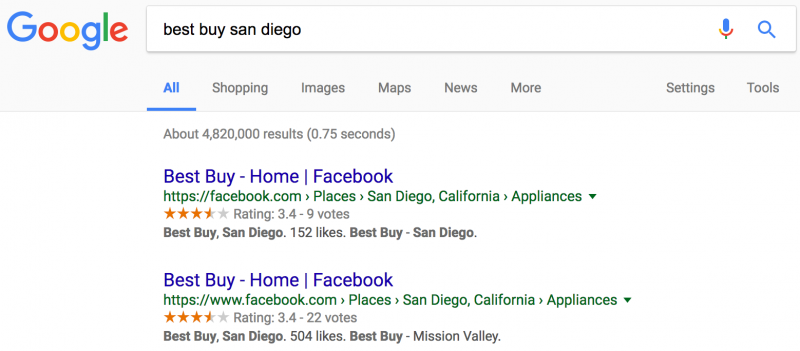This is an image of a Google search results page featuring Google's signature colors: blue, red, yellow, and green. At the top, prominently displayed, is the Google logo followed by a search bar with the query "Best Buy San Diego". Underneath the search bar, standard navigation tabs are visible: "All," "Shopping," "Images," "Maps," "News," "More," "Settings," and "Tools."

Below the tabs, a brief summary indicates that there are approximately 4,820,000 search results, retrieved in 0.75 seconds. The first search results consist of the Best Buy homepage and their Facebook page, both links appearing in blue. Specifically, the URLs are "https://facebook.com" and "Best Buy San Diego." 

The detailed information for these links includes subheadings like "Places," "San Diego, California," and "Appliances," with some rating details such as "3.4 stars from 9 votes" and "152 likes" for Best Buy San Diego. 

Further down, another result shows a Facebook page for "Best Buy Mission Valley" which has a rating of 3.4 stars from 22 votes and 405 likes. The headers for the links are in blue, while all URLs are highlighted in green. The background for the entire page is a clean, plain white.